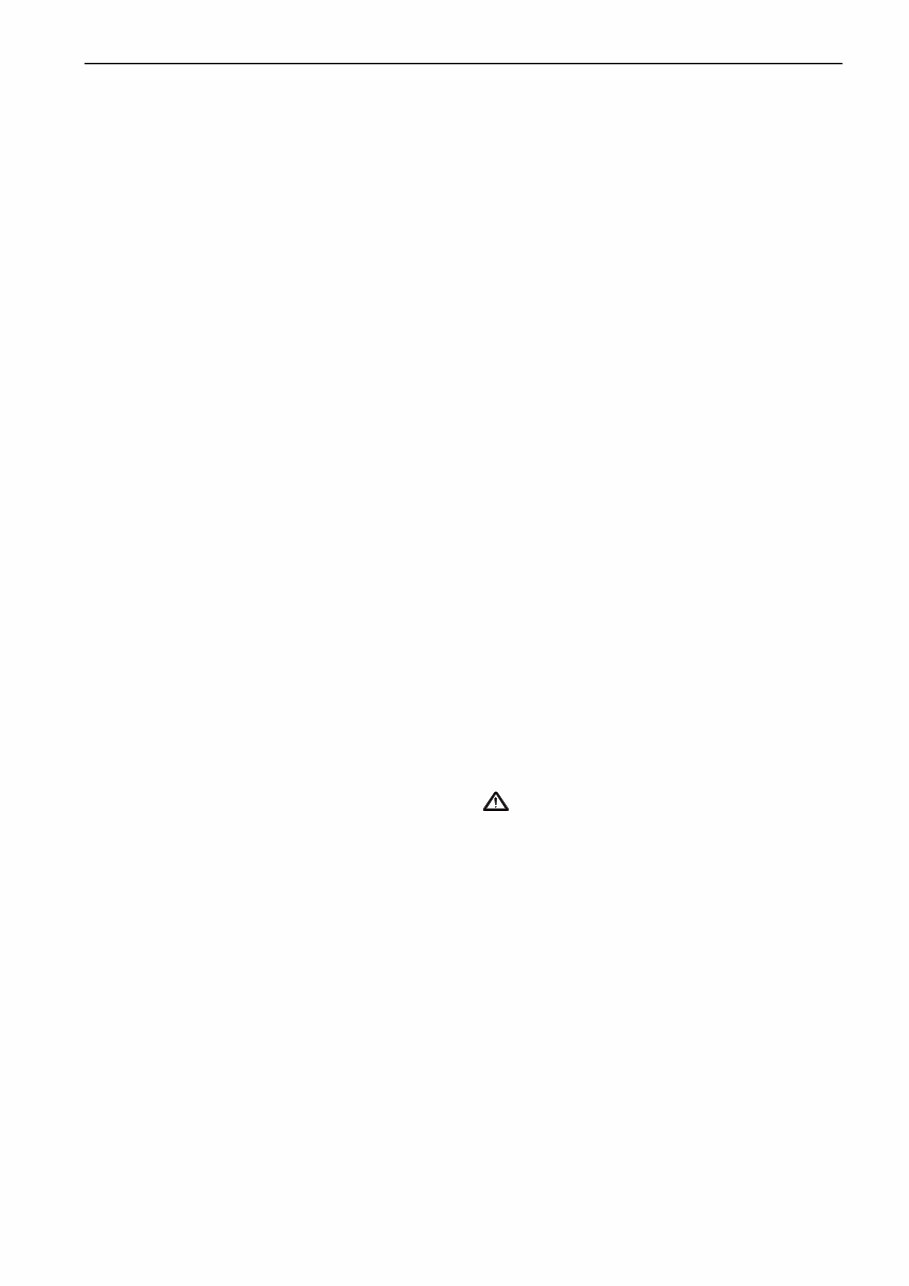The image depicts a predominantly blank white screen, signifying an absence of loaded content from the website being viewed. At the top, there is a dark horizontal line that stretches across the width of the screen. Centrally positioned, a prominent warning icon—a triangle with an exclamation point inside—stands out, indicating an error or missing content. The surrounding space remains starkly white, devoid of any images or text, emphasizing the incomplete webpage loading. The overall scene conveys an unpopulated, empty web page with a clear indication of a loading issue or error.